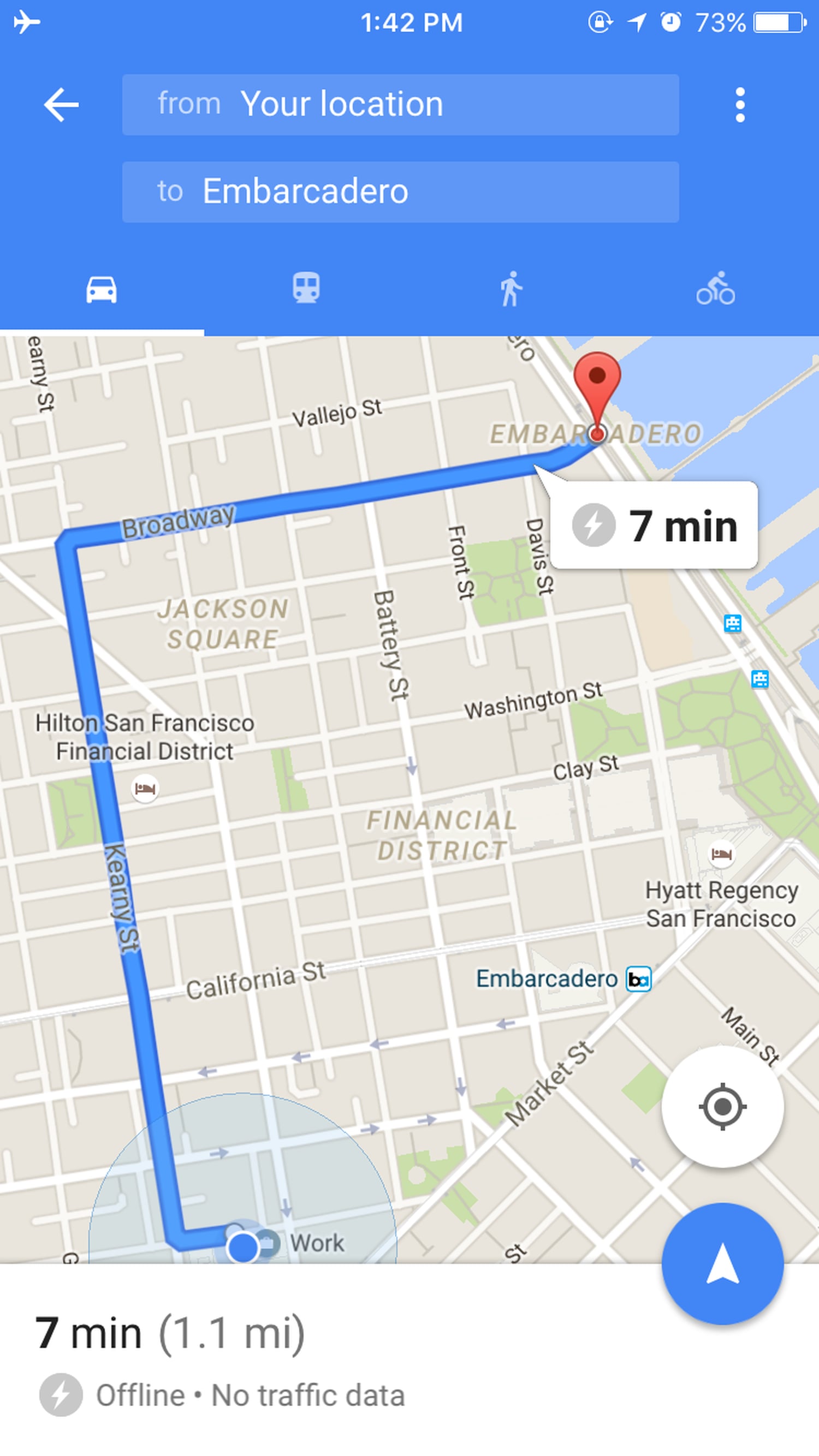The image depicts a detailed screen capture of a Google Maps navigation interface on a mobile device. The top two inches feature a light blue background, indicating the status bar and navigation options. The status bar includes various icons: an airplane mode icon on the left, followed by a battery icon showing 73%, an alarm clock icon, an upward-right arrow icon, and a circle icon indicating the screen is locked. At the center of the status bar, the time is displayed as 1:42 PM.

Below the status bar, the main interface of Google Maps is visible from the top two inches down to about an inch above the bottom, where the map is bordered by a white background. On the map, an airplane icon is located in the top-left corner. Adjacent to this icon, towards the right, there is a white arrow pointing left. Below the airplane icon, a lighter blue rectangle contains the text "From your location" in white. Underneath, another light blue rectangle reads "To EMBARCADERO."

To the right of the "From" bar, there are three vertical white dots indicating more options. Beneath these blue rectangles, a series of icons represent various modes of transportation: a car icon (highlighted with a white line underneath), a bus icon, a walking icon, and a bike icon on the far right.

The map itself occupies a significant portion of the screen. Approximately two inches from the right, a location icon is marked. Additionally, a blue route line traverses from near the left side to almost the bottom of the map, outlining the suggested directions. The map's land area is shaded gray, with some green areas representing parks, and a blue region in the upper right corner indicating a body of water.

A small white tab below the location icon displays "7 MIN" in black. In the bottom-left corner of the map, a circle indicates the location icon, beneath which is a blue circle with a white arrow pointing upward.

In the white section below the map, on the left side, "7 MIN (1.1 MI)" is prominently displayed in black text. Underneath this, a gray circle with a white lightning bolt icon appears, accompanied by the text "Offline. No traffic data."